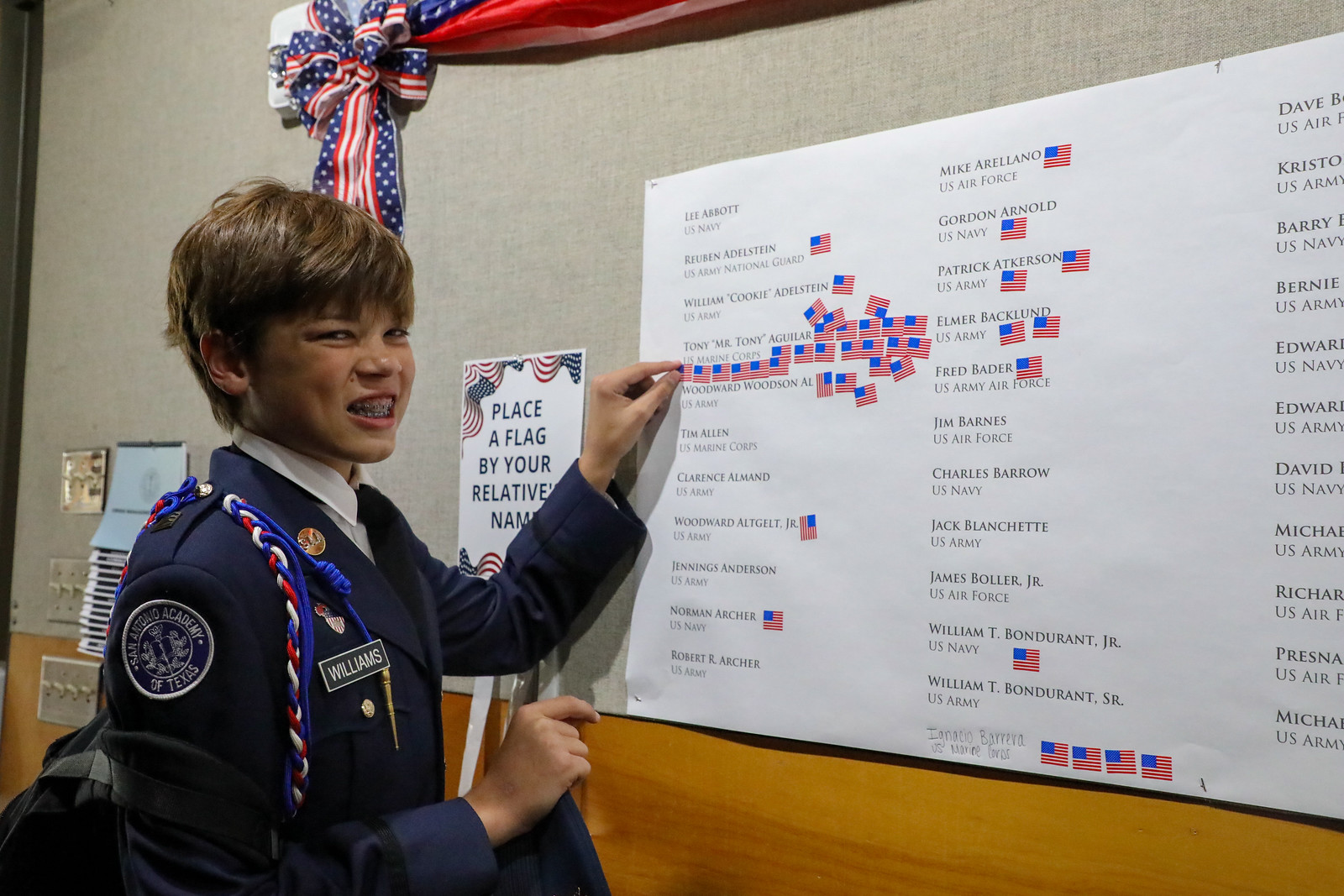The photograph captures a young boy with brown hair, dressed in a blue military-style uniform adorned with red, white, and blue strings over his shoulder and a circular red insignia patch on his right arm. A black name tag on his right lapel reads "Williams." Underneath his uniform, he wears a white shirt. The boy, sporting braces and an attempted smile with squinted eyes, is placing American flag stickers on a white board, which has various names written on it. Some names are densely covered with flag stickers, while others have none or just a few. A sign to the left of the board instructs to "place a flag by your relative's name." The board, attached to a gray thumb board, has a red, white, and blue ribbon with an American insignia in the upper left corner. Below the board is a light wooden wall, and light switches can be seen turned on in the far left corner. Behind the boy, there is a piece of paper also decorated with American flags in the top corners.